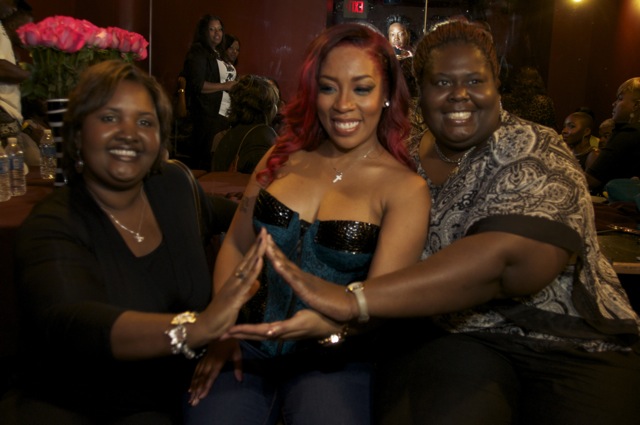This photograph captures a joyous moment of three African American women, seated together and smiling warmly as they engage in a group pose. All three women have their right hands extended to touch each other, forming a triangular shape in the center of the image. The woman on the left has short light brown hair and is dressed elegantly in a black blouse with a black cardigan. She accessorizes with a pendant necklace and a notable large silver bracelet on her right hand. The woman in the middle stands out with her long red hair. She wears a strapless blue corset adorned with black sequins, paired with blue pants, and her cross necklace adds a subtle touch to her stylish look. The woman on the right sports short dark hair and a black-and-white floral patterned blouse, also smiling radiantly. In the dimly lit background, which features red lights, the setting appears to be a lively environment like a restaurant, party, or lounge. Other people can be seen, contributing to the atmosphere. A beautiful bouquet of pink roses behind the women further enriches the scene, adding a touch of elegance and celebration.